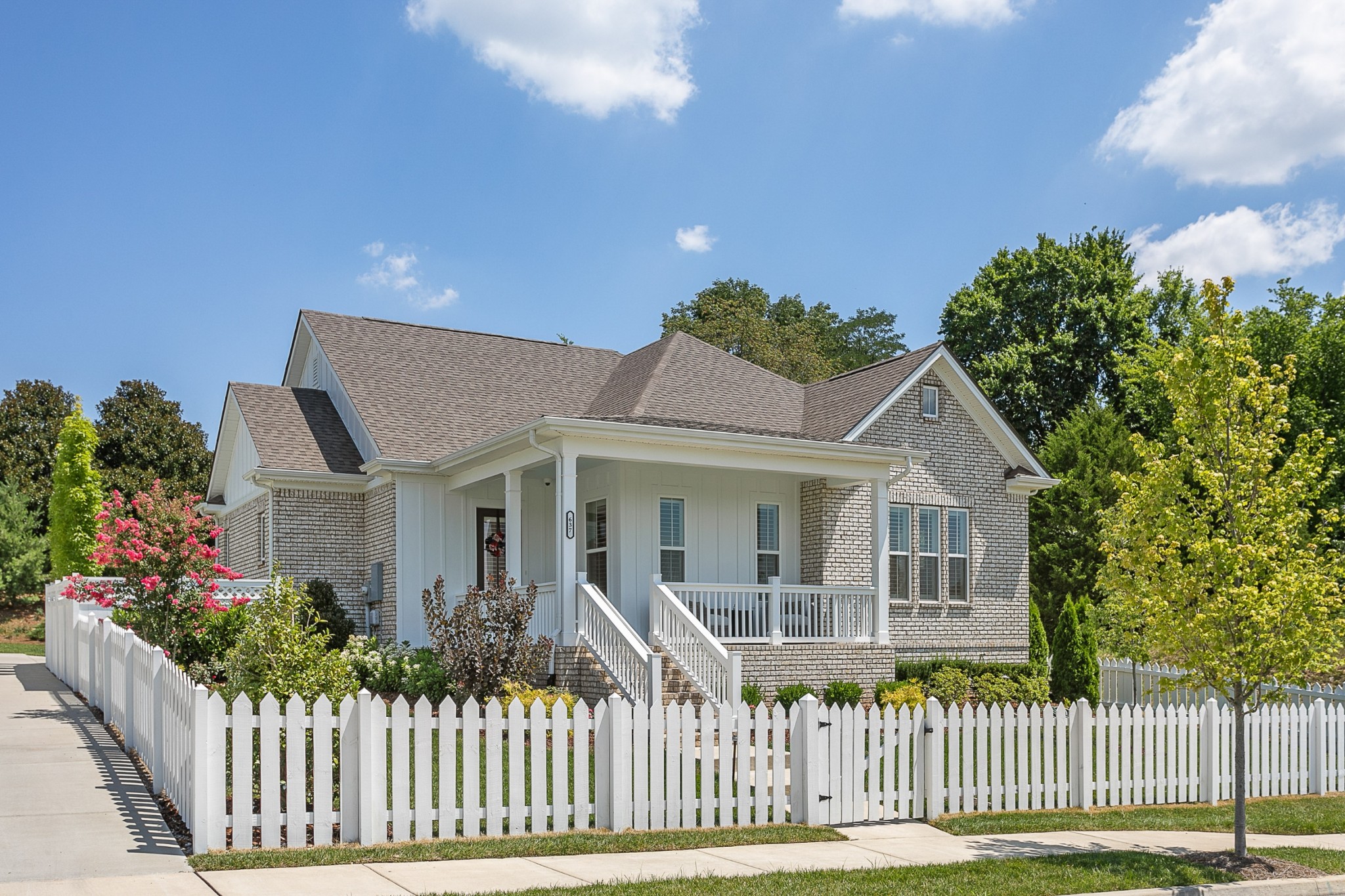This is a professional-quality photograph of a charming two-level house, possibly intended for a real estate listing. The house features a modern design with a mix of white exterior and beige and light brown brick accents. It has a shingled gray roof with a small window at the crest of the overhang. The front of the house showcases a white porch with a balcony supported by white banisters and beams, leading down to white stairs and handrails. 

Surrounding the house is a beautifully landscaped yard enclosed by a four-foot-tall white picket fence. The garden is lush with various greenery, including flowering bushes with pink blooms, dark green and light green trees, and pyramid-shaped evergreen trees. There are also some yellow and brown plants, adding a touch of color diversity. The front yard also features small green bushes and a light green plant.

In front of the fence runs a light gray sidewalk flanked by neat grassy strips. A curb is visible at the right corner of the image. Outside the gate, there is a small tree and larger trees in the background, contributing to the serene, natural setting. It's a bright and beautiful day, with a clear blue sky adorned by a few fluffy white clouds. The house number, 637, is prominently displayed, making the entire scene picturesque and inviting.